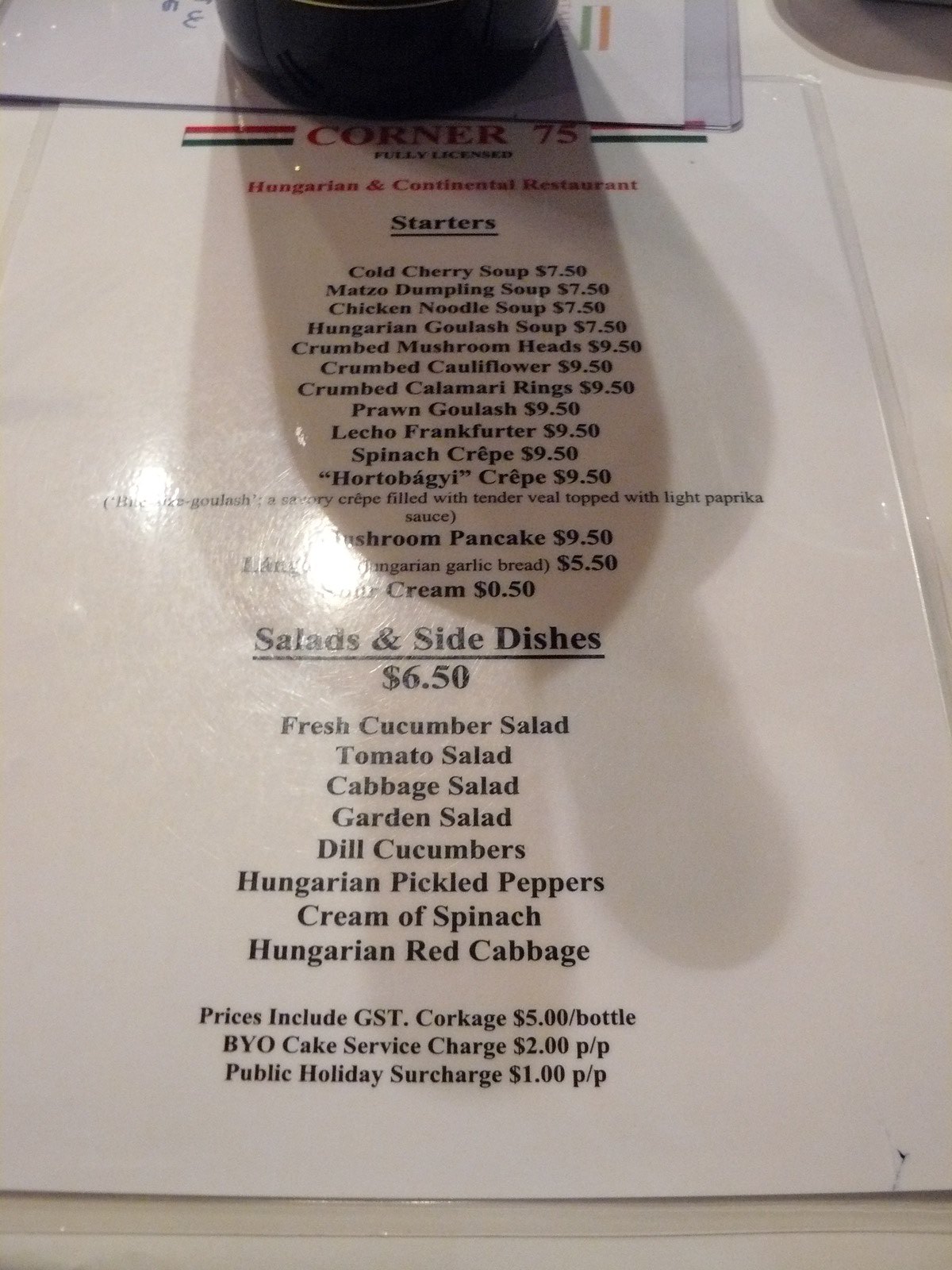This photograph captures a detailed image of a restaurant menu placed on a white tabletop, occupying most of the frame. The menu, printed on an A4-sized piece of paper and laminated, has clearly visible text along with some elements that are partially obscured by light reflections and shadows.

At the very top, the restaurant name "Corner 75" is prominently displayed in bold red font. On either side of the name, there is a flag with red, white, and green horizontal stripes. Below the restaurant name, the words "Fully Licensed" appear in black, followed by "Hungarian and Continental Restaurant" in red.

The menu begins with the "Starters" section, which is underlined for emphasis. The starters listed include:

- Cold Cherry Soup - $7.50
- Matzo Dumpling Soup - $7.50
- Chicken Noodle Soup - $7.50
- Hungarian Goulash Soup - $7.50
- Crumbed Mushroom Heads - $9.50
- Crumbed Cauliflower - $9.50
- Crumbed Calamari Rings - $9.50
- Prawn Goulash - $9.50
- Lecho Frankfurter - $9.50
- Spinach Crepe - $9.50
- Hortabagi Crepe - $9.50

A section of the text explains that Hortabagi Crepe is a savory crepe filled with tender veal, topped with a light paprika sauce.

There is a noticeable shadow across the starters section, cast by an undefined object at the top of the image, making some items less readable due to the light shining on the laminated surface.

Further down, the menu lists "Salads and Side Dishes" priced at $6.50 each, which include:

- Fresh Cucumber Salad
- Tomato Salad
- Cabbage Salad
- Garden Salad
- Dill Cucumbers
- Hungarian Pickled Peppers
- Cream of Spinach
- Hungarian Red Cabbage

Additional information at the bottom of the menu states that prices include GST. There are also notes regarding extra charges: a corkage fee of $5 per bottle, a BYO Cake Service Charge of $2 per person, and a Public Holiday Surcharge of $1 per person.

The lighting and shadows in the photograph add a dynamic element to the otherwise static image of the menu, illustrating the ambiance and setting of the dining experience.